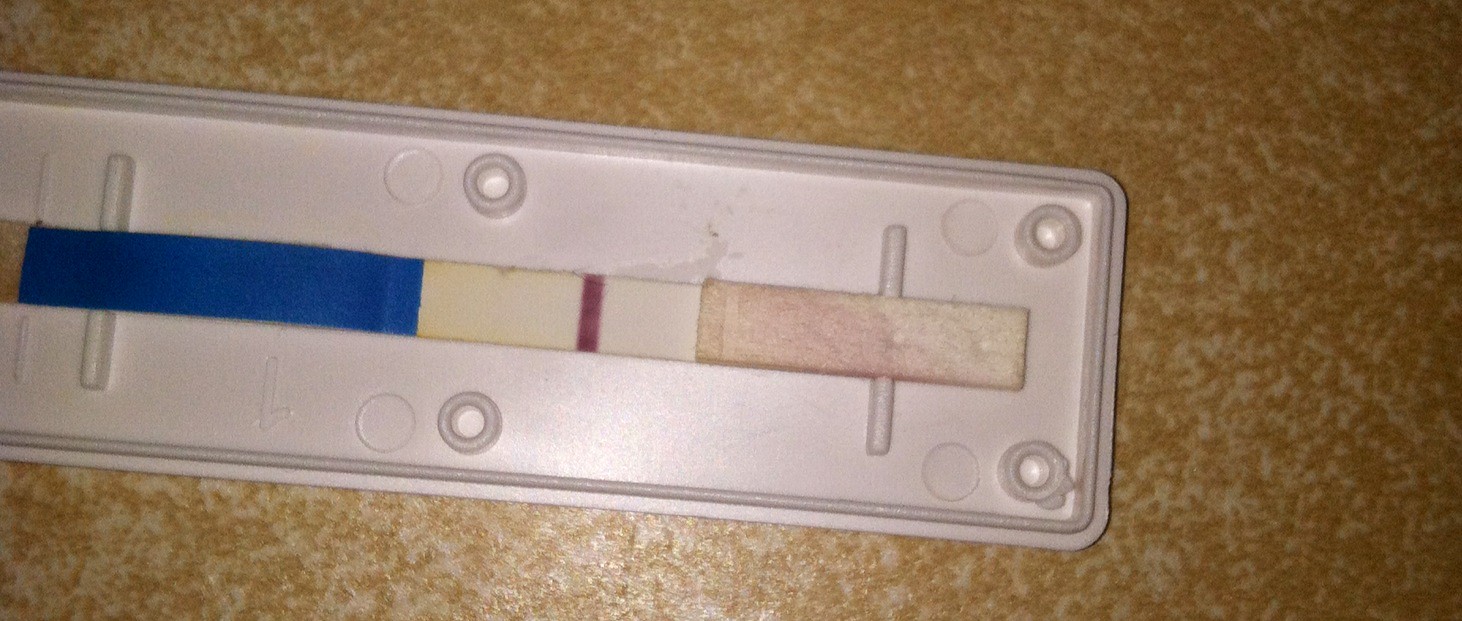The image depicts an opened COVID-19 test kit laid out on a countertop. The test kit includes a white plastic cassette that is rectangular in shape. The cassette is turned upside down, revealing its inner components. On the right side of the cassette, there is a long, white rectangular test strip. This test strip features a red vertical line on its left side, followed by a small white section, and then a long blue area towards the right. The overall assembly is indicative of a lateral flow test setup, primarily used for determining COVID-19 positivity through a swab sample applied to the test strip.